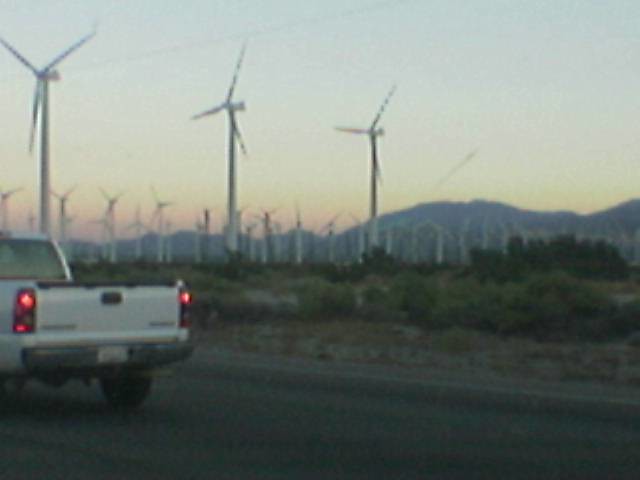This color photograph captures a serene moment just before sunset in an expansive, open landscape. The sky transitions from hues of pink and red near the horizon to a gray haze as it stretches upward. The foreground features a white pickup truck with its brake lights illuminated, positioned toward the left side as if it’s driving away. You can discern the truck's bed, rear window, and two prominently dark tires. Behind the truck lies an expansive field punctuated by dozens of massive white wind turbines, their blades slowly turning against the sky. These turbines, numbering perhaps 40 or 50, continue as far as the eye can see. The scene is set against a backdrop of softly faded hills and mountains, tinged with purples and grays that blend into the distant horizon. Sparse wires cross the sky, adding to the desolate, remote ambiance, reminiscent of a desert area being traversed.